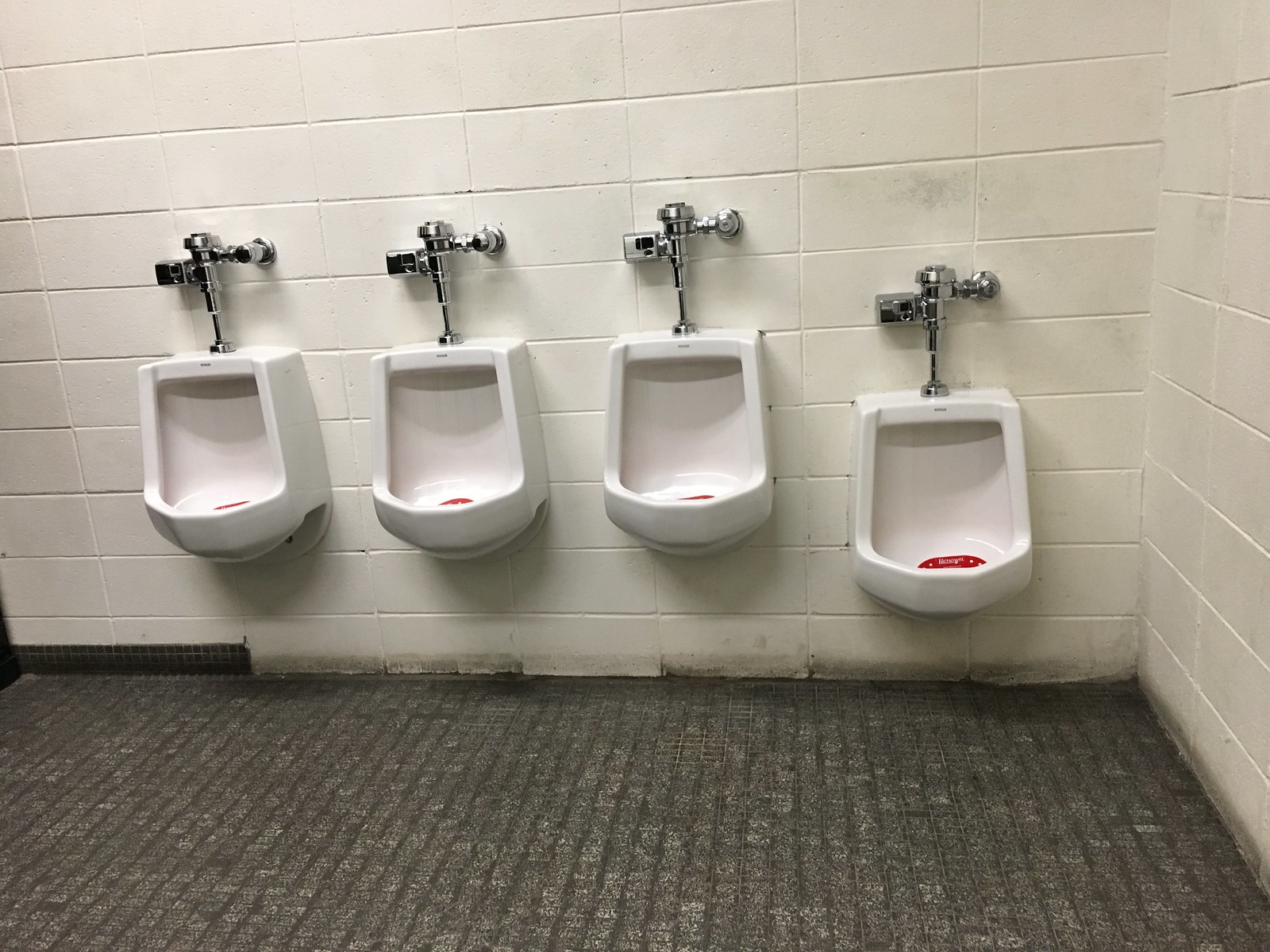The photograph depicts a men's bathroom with four urinals lined up against a concrete white brick wall. The most striking feature is the floor, which is covered in a nasty, gray carpet—an unusual choice for such a setting. The urinals are mostly of the traditional type, equipped with silver sensors that ensure automatic flushing. Notably, there is a urinal on the far right that is positioned lower than the others, designed for children. All the urinals contain red urinal cakes for freshness. A rubber baseboard runs along the bottom of the wall but ends abruptly halfway under the first urinal on the left, making it look as though it's been partially removed. The base of the wall is dirty, showing black marks and signs of wear. The general layout provides absolutely no privacy between the urinals.